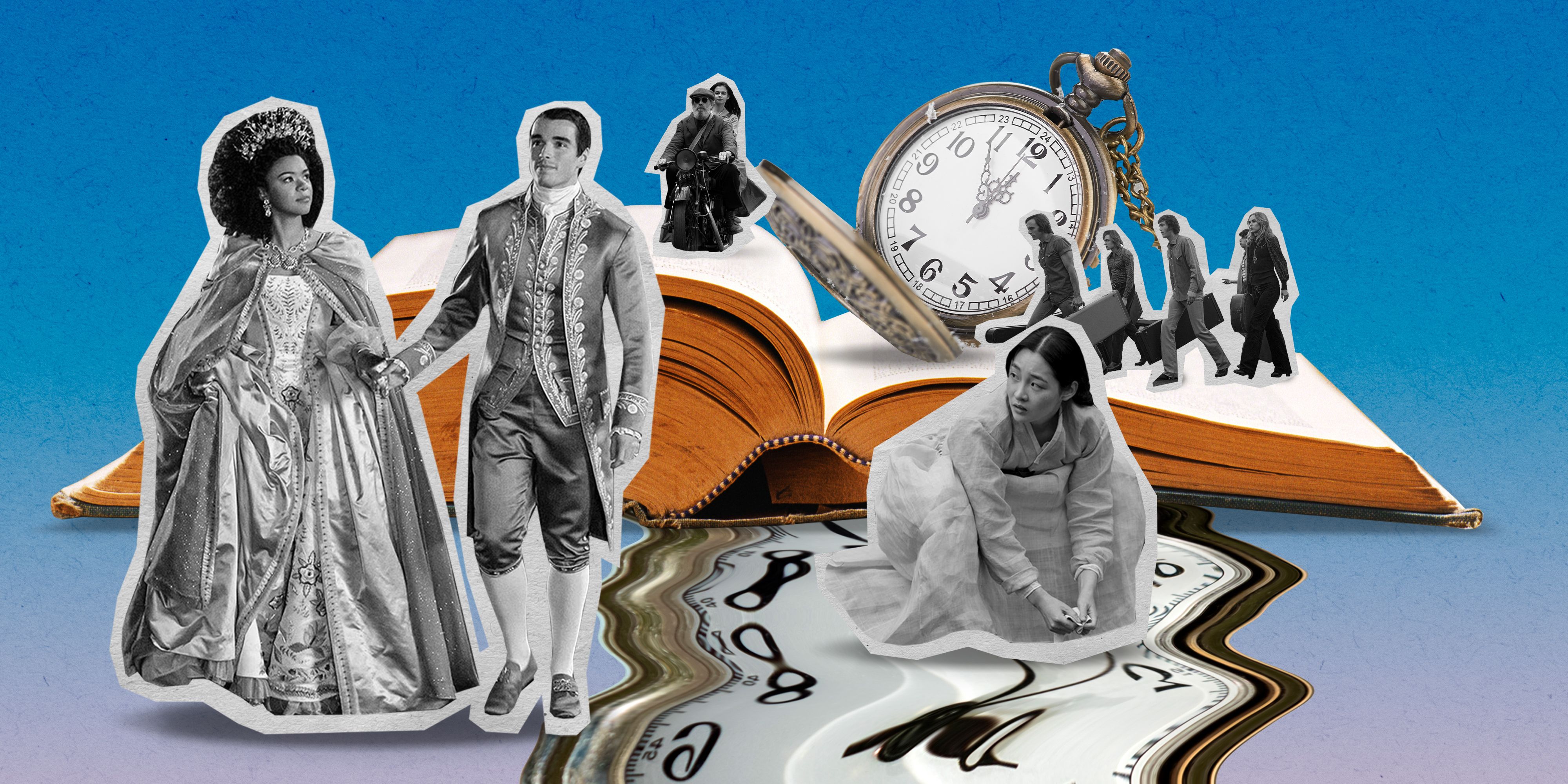The image is a detailed collage showcasing an eclectic mix of characters superimposed onto a bluish-purple background. On the left, there is a regal couple clad in Victorian clothing; the man, who appears to be a lord, is dressed in a suit, while the woman, a dark-skinned madame with African features, wears a large gown and a tiara. Moving to the right, there is a Korean woman bent over, seemingly washing over a melted analog clock whose hands are also distorted. Behind these figures, a page from an open book forms the backdrop, on which stands a group resembling 60s band members, likely The Beatles, each carrying musical instruments. To the right of this band, positioned on the same book page, is an ornate, almost midnight-striking pocket watch. Additionally, there is another couple on a motorcycle situated on the left-hand side of the book, blending seamlessly into this surreal, time-transcending scene.